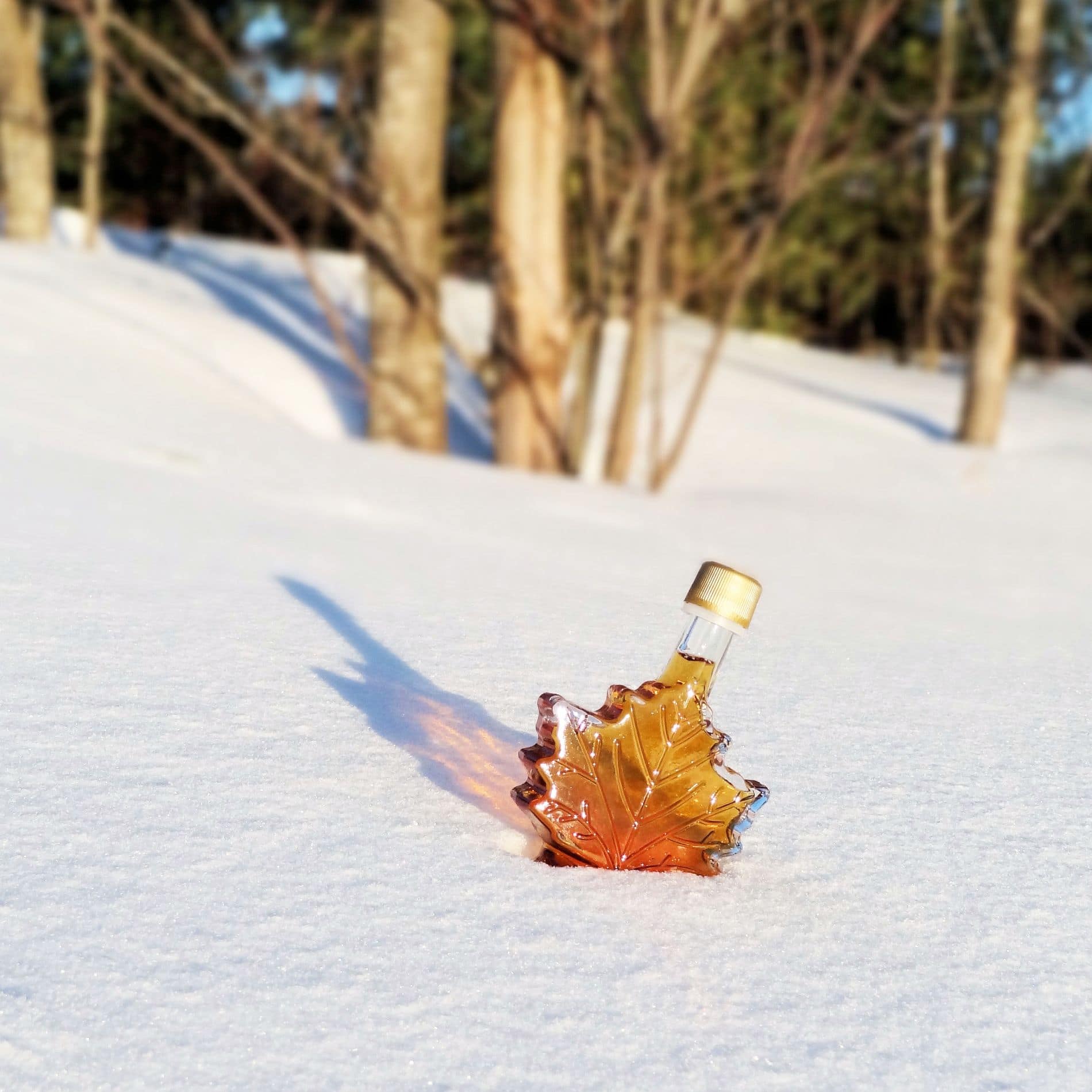This photograph depicts a stylistic and professional product image of a glass bottle shaped like a maple leaf, most likely containing maple syrup, accentuated by its amber-brown liquid. The bottle is topped with a gold-colored plastic screw cap. It is positioned upright in a pristine snow bank on what appears to be a hillside. The snow is fresh and undisturbed, with no visible footprints around the bottle, adding a sense of mystery as if it had fallen from the sky or a tree. The bottle casts a clear shadow in the snow, highlighting its unique shape. In the blurred background, several bare tree trunks, likely a mix of birch and pine, stand against the backdrop of a quiet winter forest. The overall scene is serene and picturesque, offering a striking contrast between the warmth of the maple syrup and the cold, crisp snow.